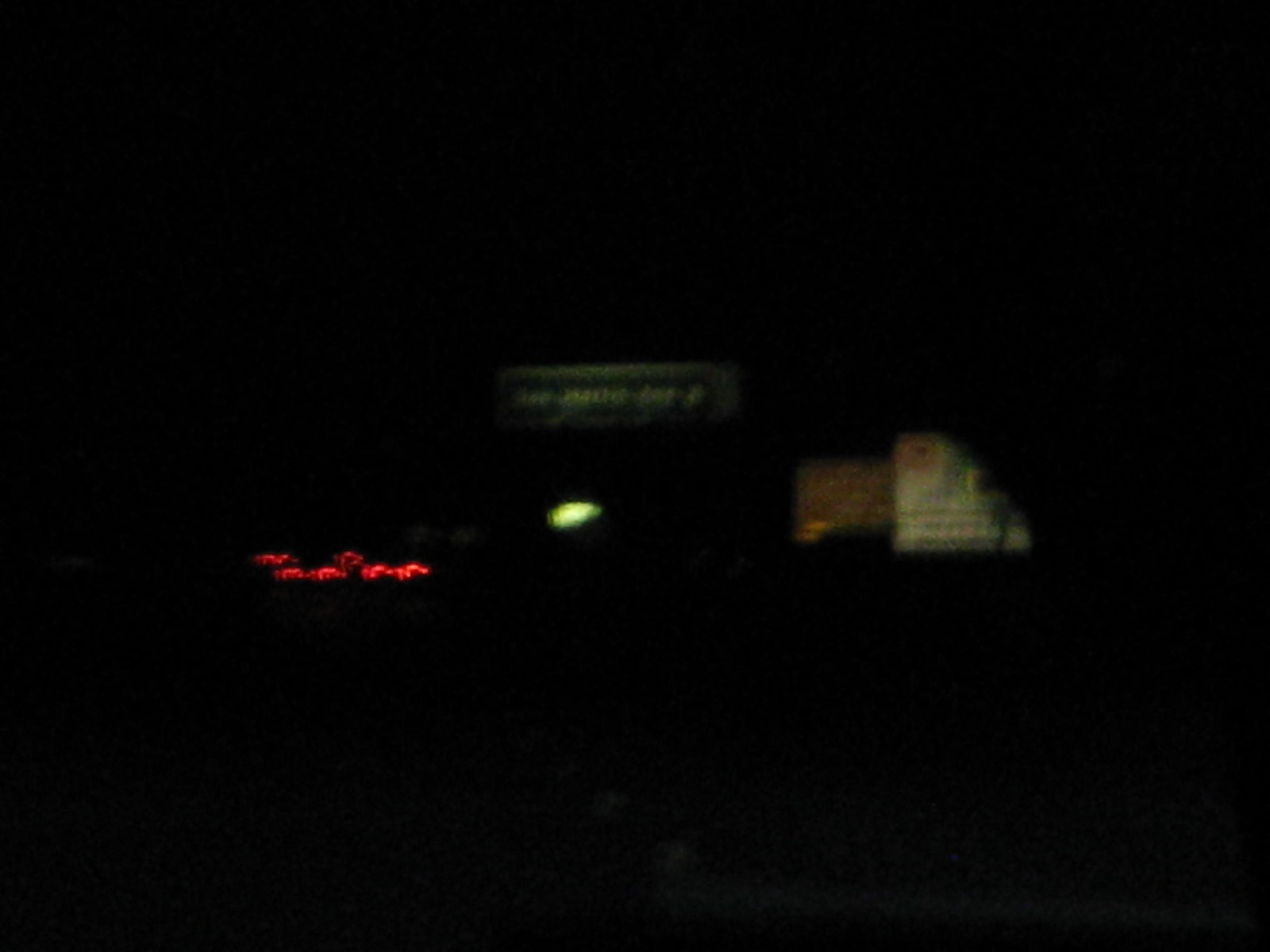The image appears to be taken from inside a vehicle at night, capturing a very blurry and dark scene. On the left side, two sets of faint taillights are barely visible, suggesting the presence of vehicles ahead. To the right, there is an indistinct billboard sign. An overpass might be present, indicated by a green street sign overhead, though its text is unreadable. Additionally, a solitary yellow light is visible, which could be the moon descending. The rest of the image is enveloped in darkness, offering no further discernible details.